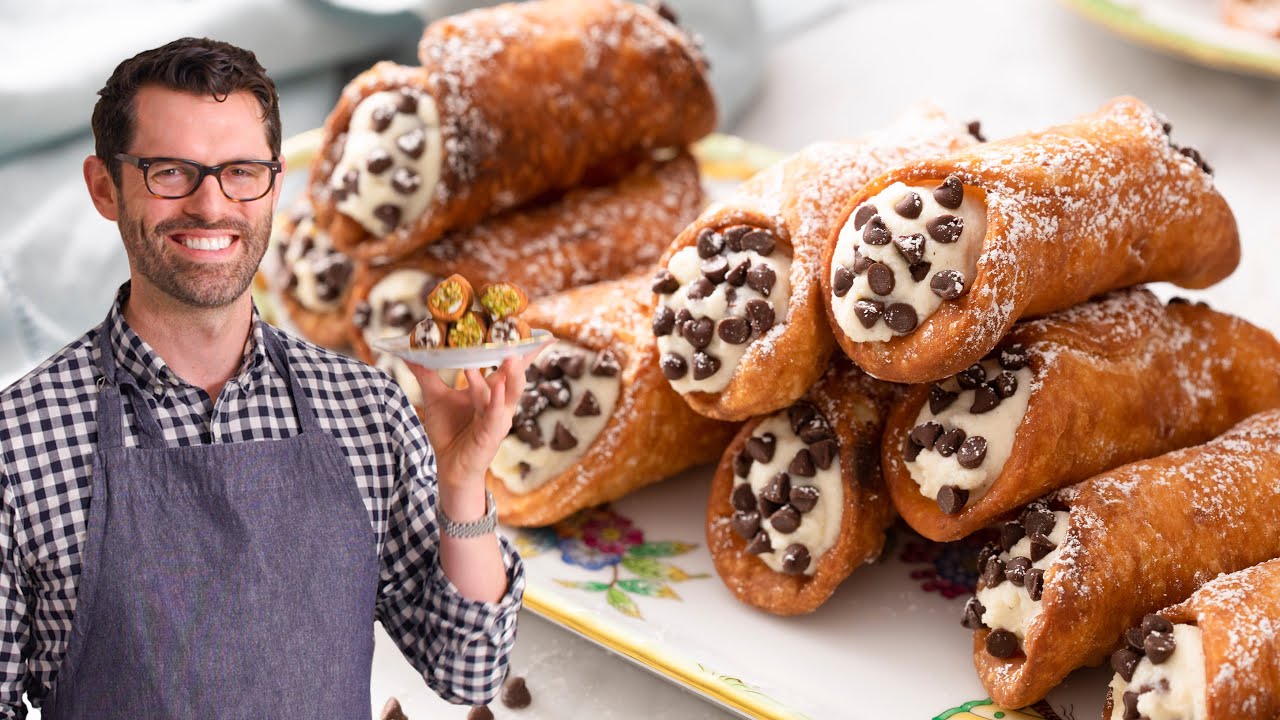In the image, a delectable stack of golden brown cannolis is set on a decorative white porcelain platter, delicately outlined in gold, with a multicolor flower design peeking through from the covered parts. The cannolis are generously dusted with powdered sugar, and the creamy white filling inside is embellished with chocolate chips. At least ten cannolis are piled on the platter. On the left side of the image, a man with wavy brown hair, donning a neatly trimmed beard and mustache, is holding a smaller white plate with five cannolis. Some of these cannolis have chocolate chips while others are coated with what appears to be greenish-yellow pistachio nuts. The man is dressed in a black and white checkered shirt layered with a gray apron, and he wears black-framed glasses. He smiles warmly at the camera, displaying a watch on his left wrist as he raises the plate of cannolis. The set scene rests on a white table in the background.